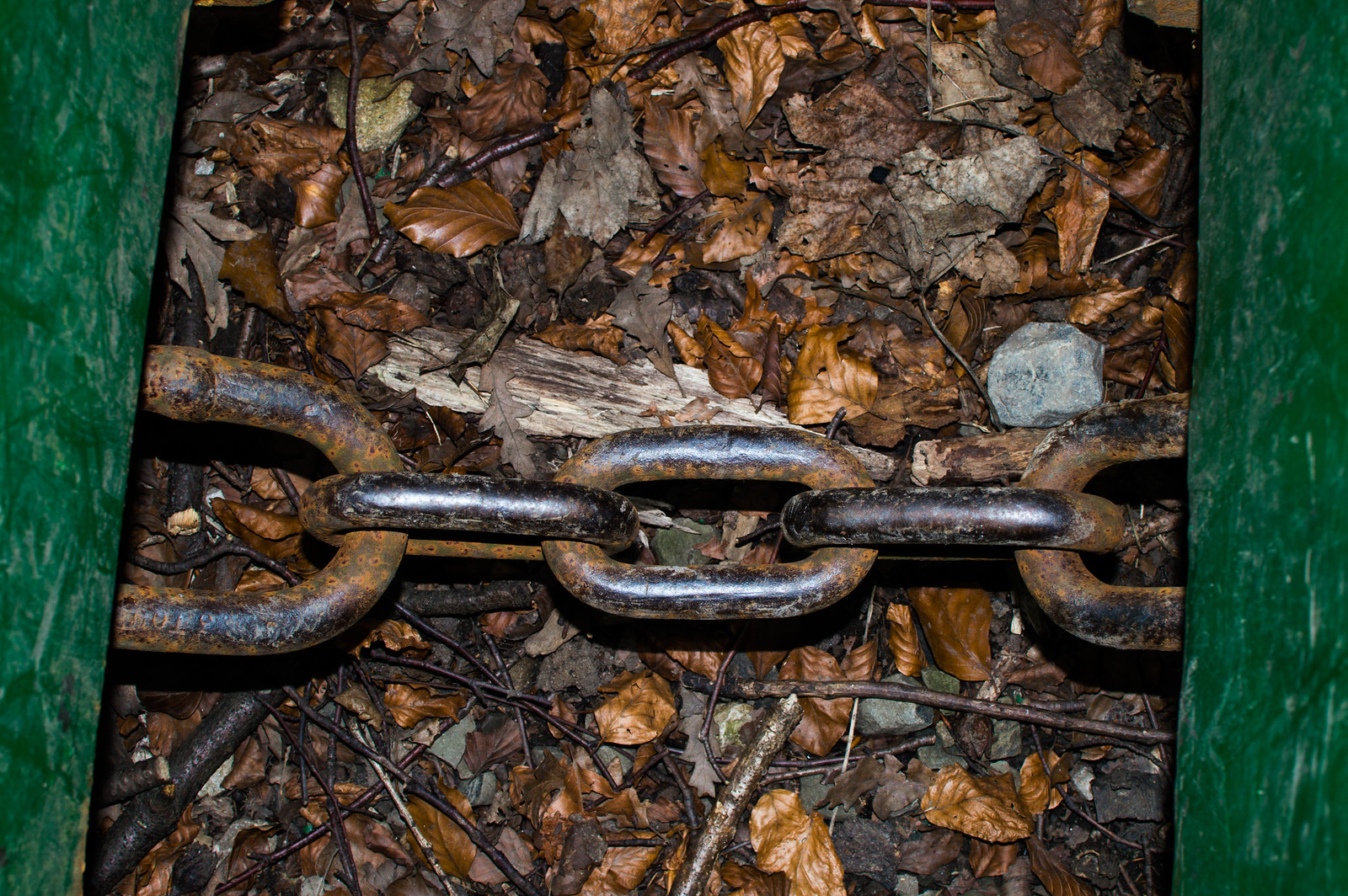A close-up image features a heavily rusted black chain with five links, connecting two vertical green planks of wood situated on the left and right sides of the picture. The chain, lying on the ground, appears both black and brown due to the rust forming on its surface. Surrounding the chain, the ground is reminiscent of a forest floor, littered with an array of leaves, including brown, gray, and black ones, as well as tiny branches and mulch. A small gray rock is noticeable atop the chain on the right side of the image. The scene gives an impression of an old, neglected connection between the two green planks amidst a natural, somewhat decayed environment.